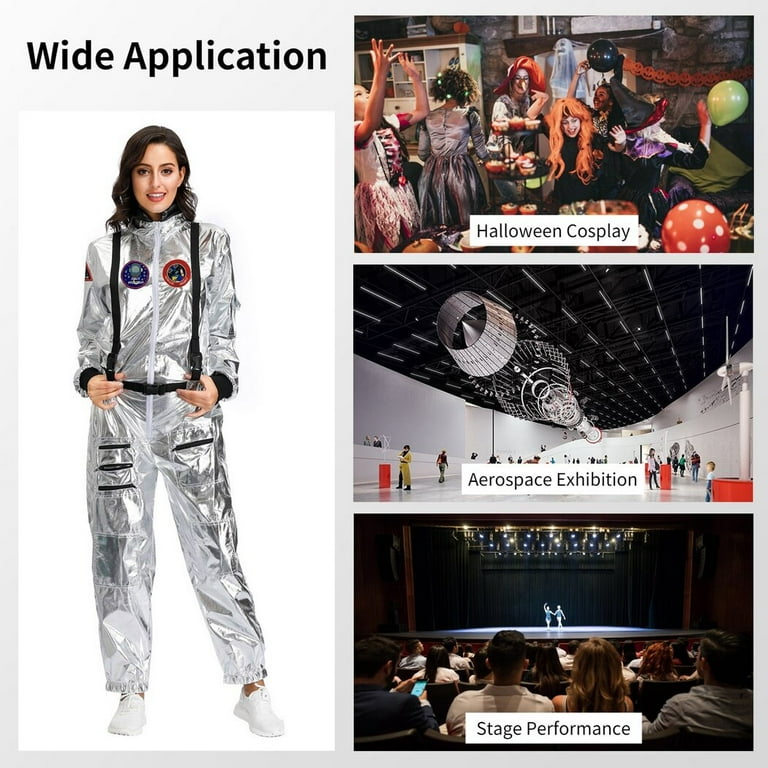This image is a collage illustrating the versatility of a silver space-themed costume worn by a young woman with shoulder-length dark hair. On the left third of the collage, against a gray background, a banner reads "Wide Application." The woman, dressed in a silver outfit with black details and patches along with suspenders, stands confidently, gazing at the camera. To the right, the collage presents three scenarios where this costume is apt. The first image, labeled "Halloween Cosplay," depicts a lively costume party featuring guests in varied outfits, including bright orange wigs and witches' hats, amidst floating balloons. The second image, titled "Aerospace Exhibition," captures a museum scene with white walls, a black ceiling, and a large metallic structure overhead. Red modular tables scattered throughout hold exhibits, while attendees explore the displays. The final image, "Stage Performance," shows the backs of an audience seated before a stage lit with spotlights, where two actors, possibly ballet dancers, perform. This collage effectively showcases the costume’s adaptability for Halloween parties, museum exhibitions, and theatrical performances.